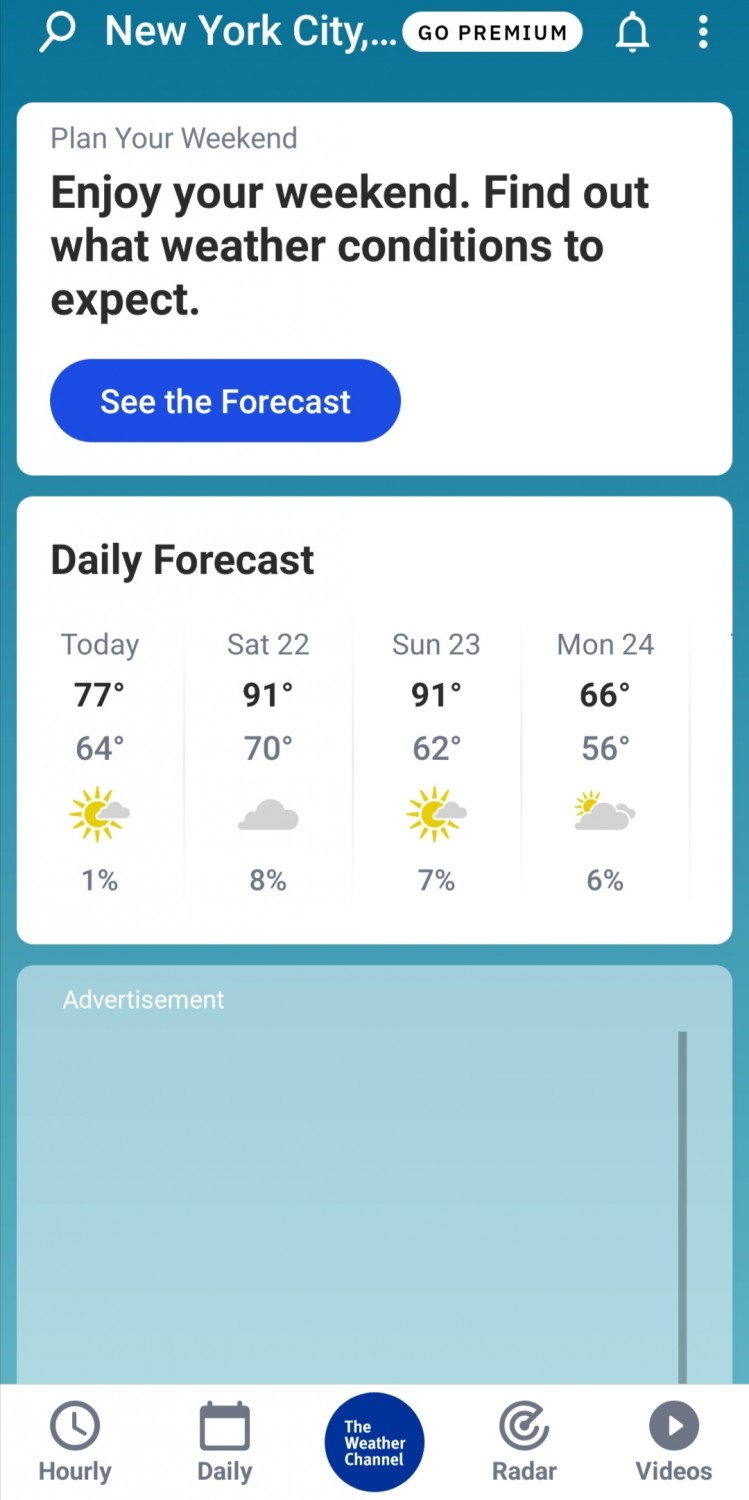The image depicts a weather app interface on a mobile phone, characterized by a teal background. At the top, there is a magnifying glass icon for search functionality, indicating that the current location is New York City. Adjacent to it is a white button labeled "Go Premium," suggesting the availability of an advanced, purchasable version of the app. Next to it, a bell icon is outlined in white, presumably for sending notifications, followed by a vertical ellipsis (three dots), which likely opens a hidden menu for additional features.

Beneath this header is a prominent white box containing the text: "Plan your weekend, enjoy your weekend, find out what weather conditions to expect." Directly below this text is an oblong blue button with white text that reads "See the forecast," indicating that tapping it will display the weather forecast for New York City.

The next section provides a detailed daily forecast in a structured format, featuring columns for each day. Each column shows the high and low temperatures along with an icon representing sky conditions, such as partly cloudy, cloudy, or mostly sunny. Below each sky condition icon is the percentage chance of rain for that day.